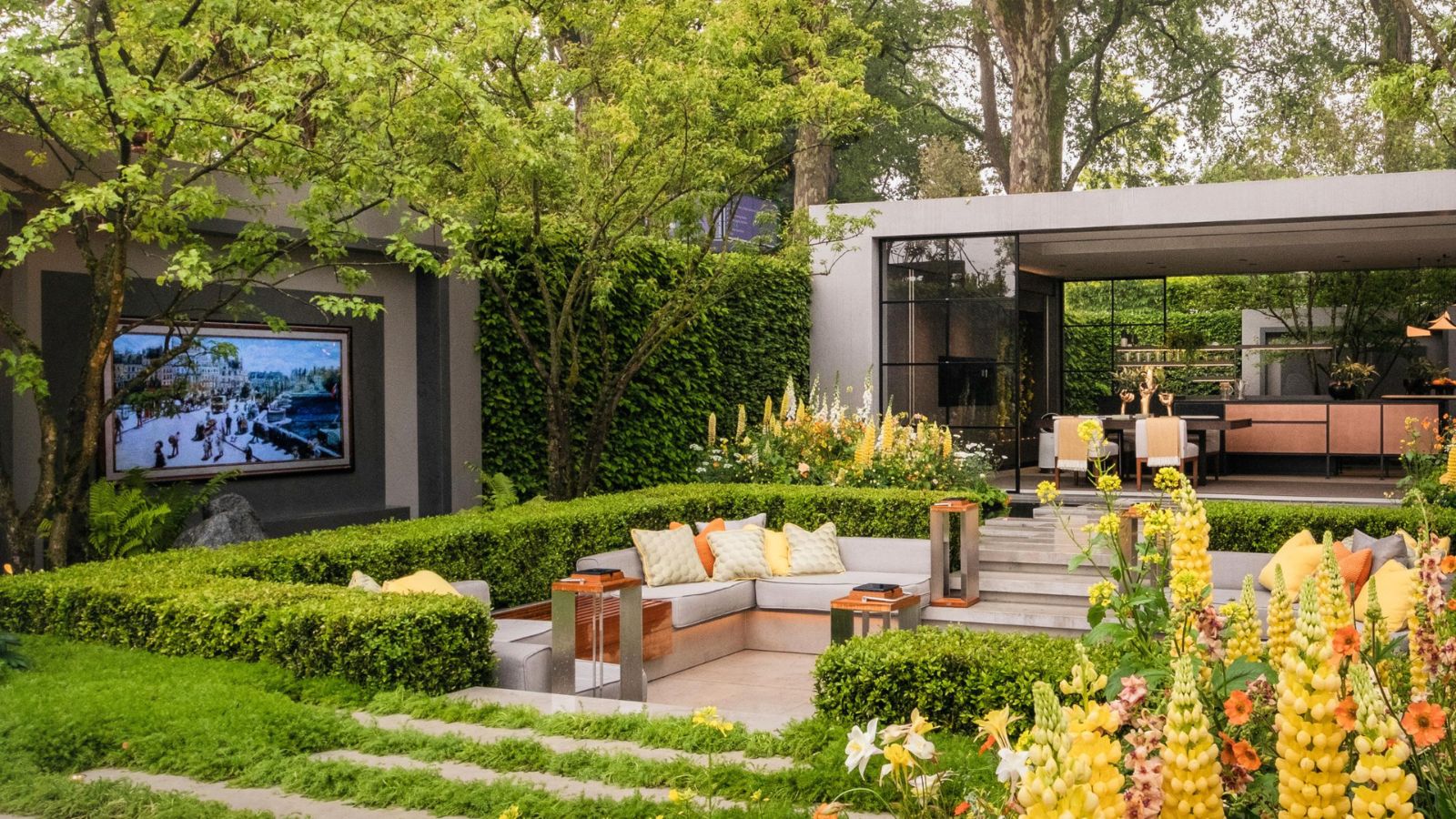The image features a luxurious multi-million dollar house with an expansive garden. The house boasts a sleek, expensive glass window on its side, offering a glimpse into its opulence. The garden is meticulously manicured, with lush green bushes and clusters of elegant yellow flowers that add a fresh, citrusy vibe to the scene. There are also other kinds of flowers, including white ones growing upwards. Outdoor furniture is arranged on a rectangular cement patio, which includes gray couches adorned with pillows, adding a touch of comfort and style. The patio also features areas for cooking, lighting, and seating with chairs and tables. Stairs lead down from the patio, which is bordered by cement pillars. In the left-hand side of the image, a TV monitor is visible, adding to the modern amenities of this outdoor space. The background is filled with towering trees and a bright sky, enhancing the serene atmosphere of this beautifully maintained garden.